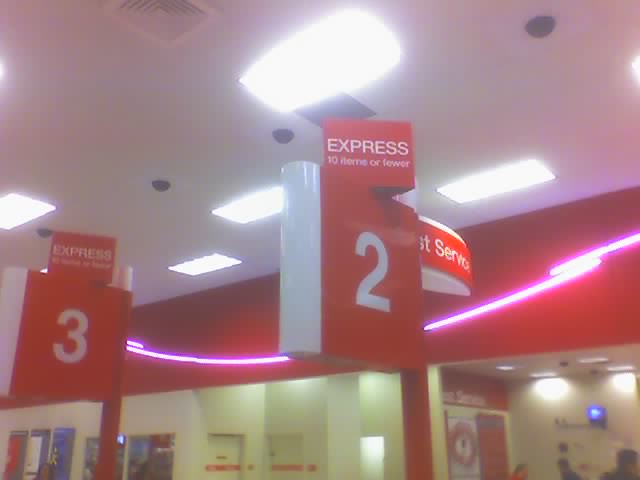This indoor photograph appears to be taken in a Target store, focusing on the checkout area. The image prominently features the express lanes, marked by red signs with white text indicating "Express" and "10 items or fewer." Visible lanes are numbered two and three. The checkout signs, which are white, are not lit. 

A white ceiling with bright rectangular lights illuminates the area, and four security cameras are visible near the top center of the photo. A conspicuous red banner with red neon lights, resembling lightning bolts, intersects the ceiling perpendicularly. Below the banner, a tan wall hosts various advertisements and outcoves for customer service, including the two bathrooms, identified by the red door on the wall. 

Visible against the back wall, there is a blue light. Additional features along the wall include items such as a key-making station, an ATM machine, and a coin exchange machine. Finally, at the bottom right corner of the photograph, a man's head is partially visible; he appears to be wearing a black shirt.